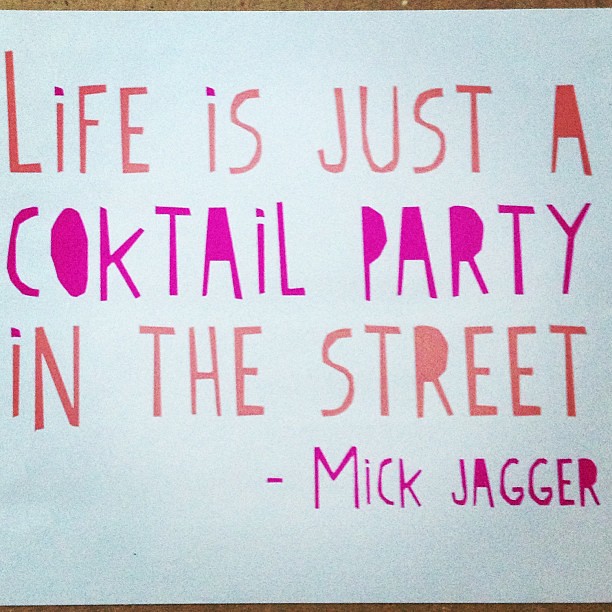This is a square image of a hand-crafted poster featuring a famous quote by Mick Jagger, displayed on a light brown surface. The poster is printed on white paper, with the edges visible at both the top and bottom. The sign begins with the phrase "life is just a" in peach-colored font, distinguished by pink dots in the letters 'i'. The prominent middle line, "cocktail party," is styled in bright pink, notably with the enclosed parts of letters like 'O', 'A', 'P', and 'R' filled in, adding a unique touch to the design. Below this, the phrase "in the street" returns to the peach-colored font. In the bottom right corner, the quote is attributed to "Mick Jagger," written in the same bright pink font with filled-in letters, separated by a hyphen. This poster captures both the aesthetic elements and the inspirational essence of Jagger’s words.